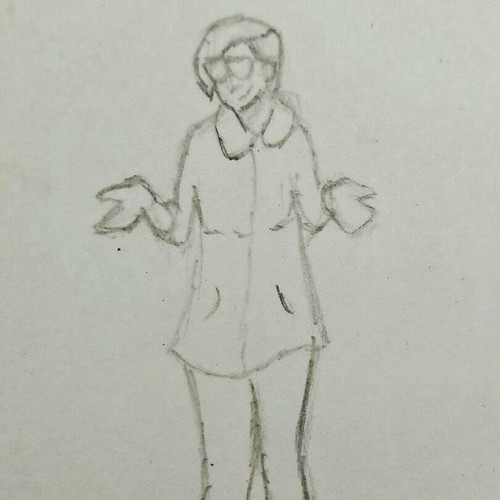This vertical, rectangular pencil sketch is drawn on slightly aged, cream-colored paper, which may appear light gray. The sole subject of the sketch is a woman whose form is cropped just below the knees and extends to the top of her head. Highlighted by a lack of color, the woman is depicted in a long-sleeve jacket that reaches her hips. The jacket features a rounded collar, a seam down the center, and small, curved lines in the lower corners suggesting pockets. Her arms are bent at the elbows with hands held out to the sides in a gesture resembling an expression of confusion or uncertainty. Her hands are drawn without distinct fingers, appearing mitten-like with a separate thumb. She is clad in pants, and her short hair is styled with a side part to her right, complemented by large glasses. The paper's off-white tone and the minimalistic nature of the sketch emphasize the simplicity and directness of the drawing.